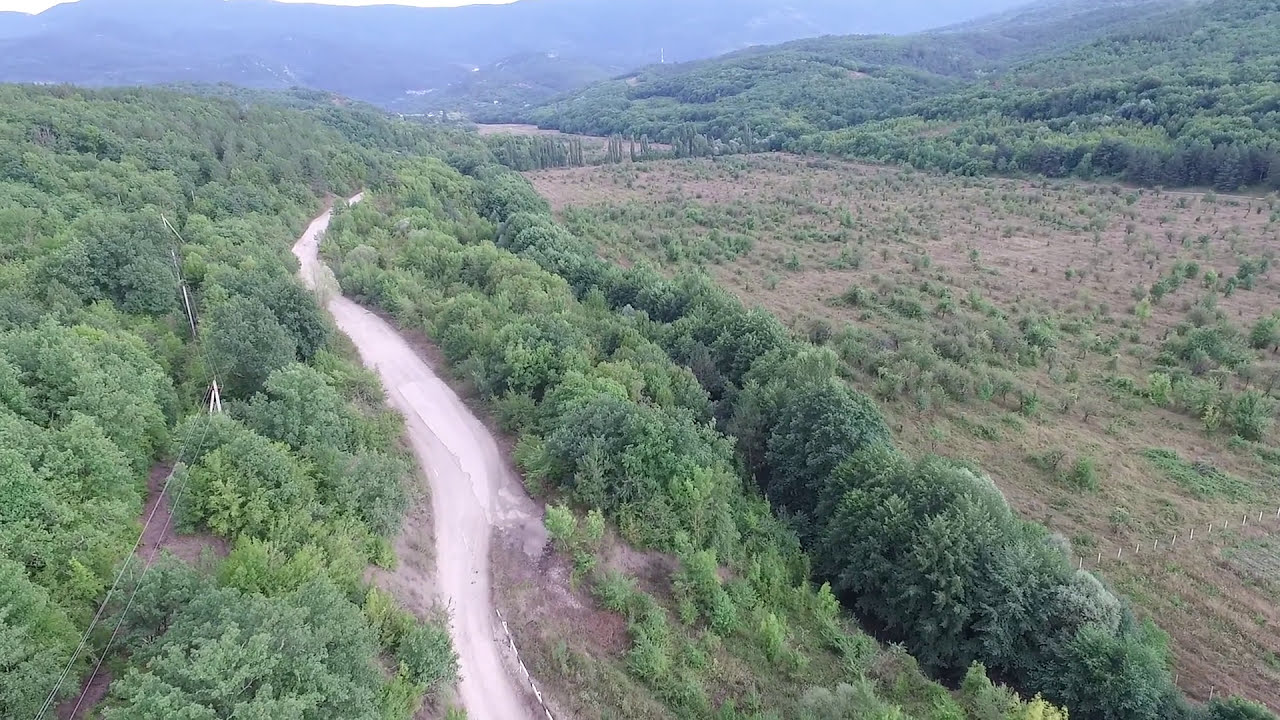In this aerial view of a countryside landscape, the sky at the top of the image is a blend of dark and light gray tones, overcast and devoid of visible clouds, casting a muted light across the scene. Dominating the upper portion of the image are multiple rolling hills, lush with green trees and shrubbery, mostly short, creating a vibrant sea of foliage. Nestled among these hills, a large white antenna stands prominently. Directly below the hills, a tidy, square farm plot, dotted with trees, is bordered by a dirt road. This unpaved road, with a washed-out appearance, winds its way from the bottom left of the image and angles towards the left, disappearing into the dense greenery. Adjacent to this road is a white and black road rail. To the left of the road, a set of double-lined power lines runs through a wooded area, their skinny poles indicative of a rural locale. On the road’s right side, a previously plowed but now somewhat overgrown field stretches parallel to the road, gradually merging with scattered bushes and trees. Encompassing both the left and right of the landscape are lush woodlands interspersed with some purplish-brown vegetation, adding a rich palette to the scene. In the distant background, the hazy silhouette of hills or mountains reaches towards the horizon, shrouded in mist, lending a tranquil and ethereal quality to this serene, uninhabited vista.